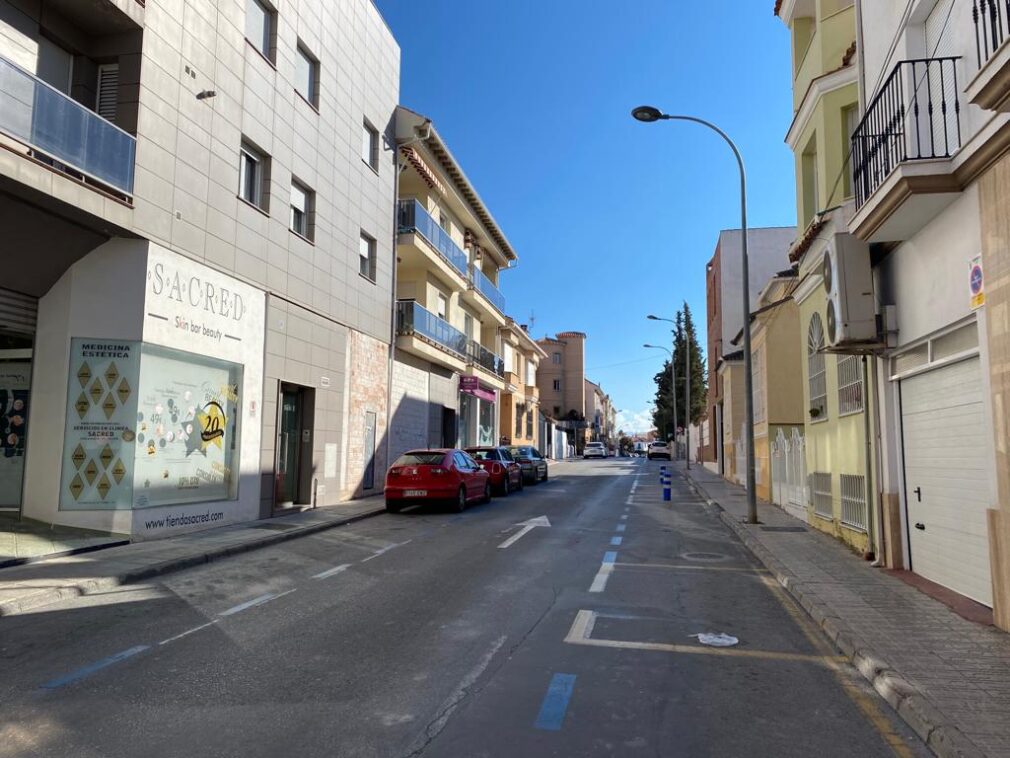The photograph captures a quiet one-way street scene, taken from a slightly right-of-center perspective. The foreground features a street arrow indicating the one-way direction, leading the eye down the length of the street. On the left side of the street, there are three parked cars: two red ones and a grayish or possibly green car. Farther down, additional vehicles are visible, parked on both sides of the street. Prominently on the left, a beauty shop called "Sacred Skin Bar Beauty" can be seen, with some advertisements displayed in the window front and possibly a web address below. The buildings lining the street showcase a range of colors, from grayish tones to hints of yellow, and are adorned with balconies, red-tiled roofs, barred windows, and streetlights. On the right side of the street, a building features a pull-in garage and an outdoor condenser fan. The sky above is clear and blue, complementing the greenery of trees visible farther down the street, suggesting a serene early morning setting. In the far background, there is a hint of a wooded area or perhaps a distant square, adding depth to the urban landscape.